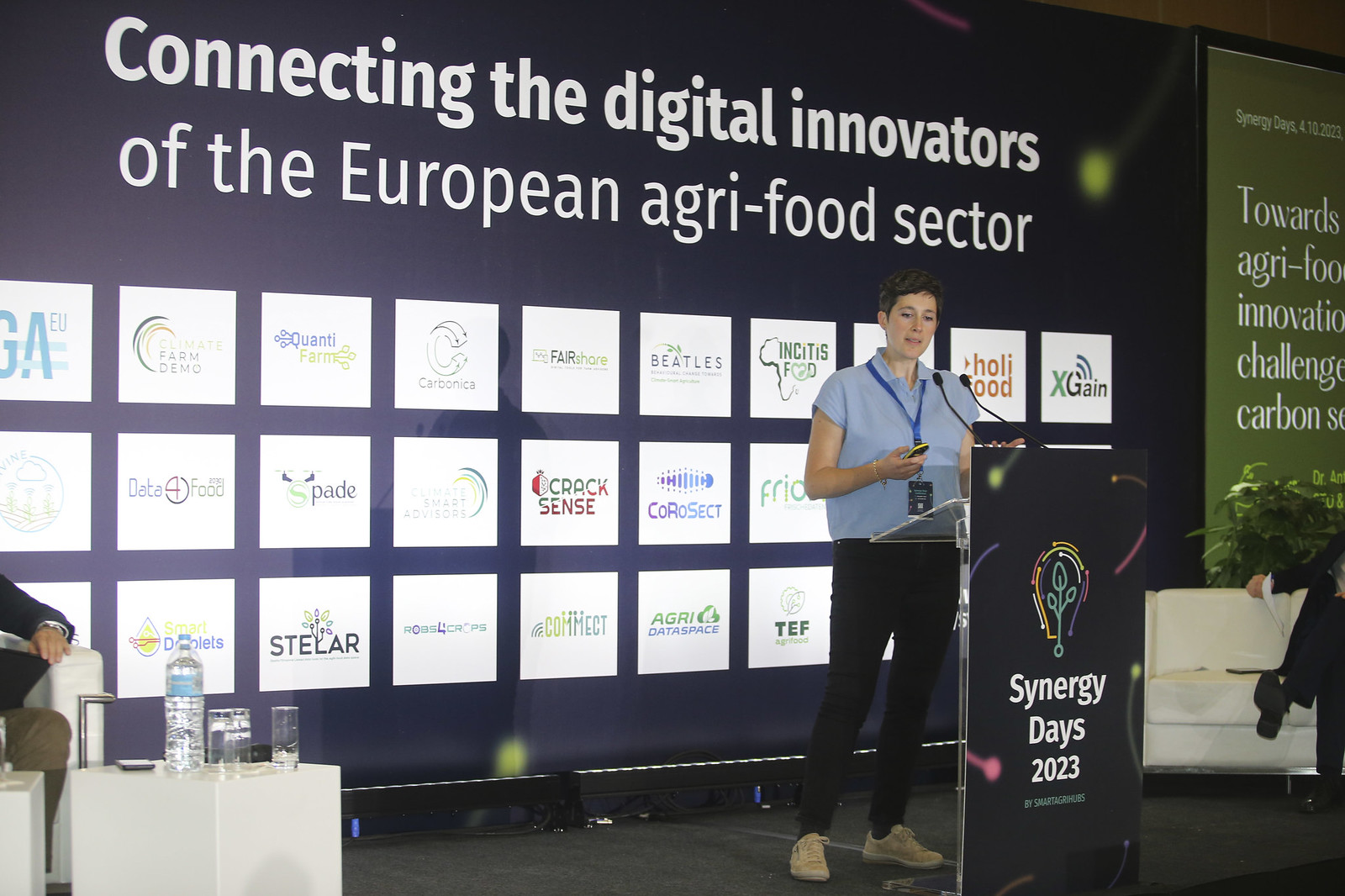The image captures a rectangular, horizontally-aligned photograph of a woman addressing an audience at a conference titled "Connecting the Digital Innovators of the European Agri-Food Sector." She stands behind a podium labeled "Synergy Days 2023," speaking into a microphone and holding a white and yellow object. The woman is dressed in a light blue, short-sleeve, collared polo shirt paired with dark pants and light tan sneakers, and she has a badge hanging around her neck. She has short brown hair.

The background features a large banner with the conference title prominently displayed and numerous white squares with company logos and sponsors' names. To the right of this banner, another banner with a green background contains partially visible words such as "Towards Agri-Food," "Innovate," "Challenge," and "Carbon."

The setting includes additional elements like a white sofa on the lower right corner, where a man is seated, his shoes and suit pants visible. Another sofa is located on the left corner with a man seated, partially obscured by the photo's edge. In front of the man on the left, there is a small white table holding a bottle of water and some drinking glasses.